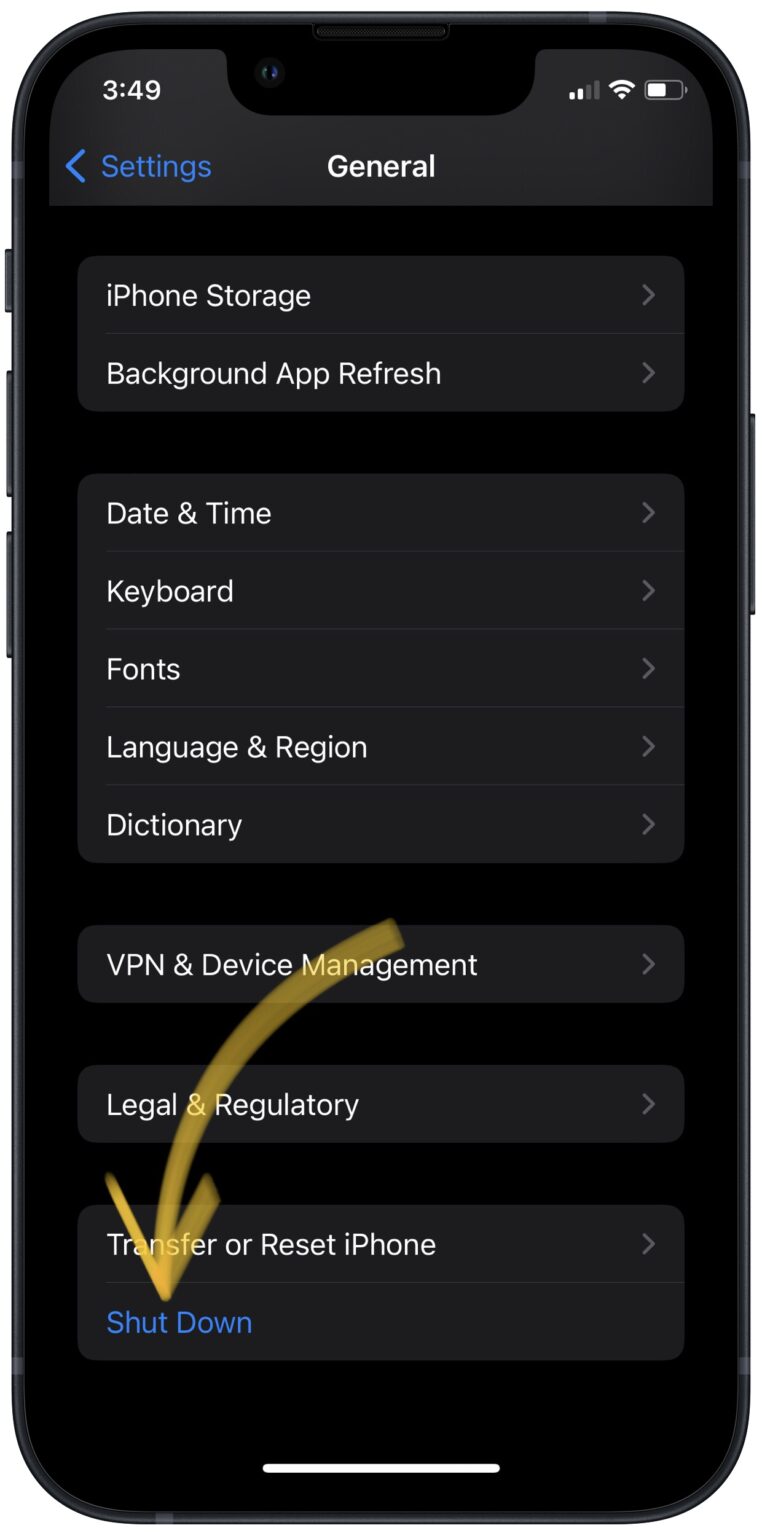The image depicts a high-resolution, close-up view of a black cell phone, prominently displayed as it might appear on an e-commerce website. The screen of the phone features a grayscale display with black accents delineating various sections. The phone is on the "Settings" page, which is identified by a blue "Settings" label in the top-left corner, accompanied by a left-facing arrow. To the right of this label, the word "General" is displayed.

The screen showcases a list of settings options, arranged vertically. The visible options include:
- iPhone Storage
- Background App Refresh
- Date & Time
- Keyboard
- Fonts
- Language & Region
- Dictionary
- VPN & Device Management
- Legal & Regulatory
- Transfer or Reset iPhone

At the bottom right of the screen, the word "Shut Down" is highlighted in blue. From the middle of the phone, a yellow arrow curves leftwards and downwards, pointing directly at the "Shut Down" label, seemingly directing the viewer's attention to this option. Additionally, a thin, white horizontal line is visible at the very bottom of the screen, indicating a navigation feature.